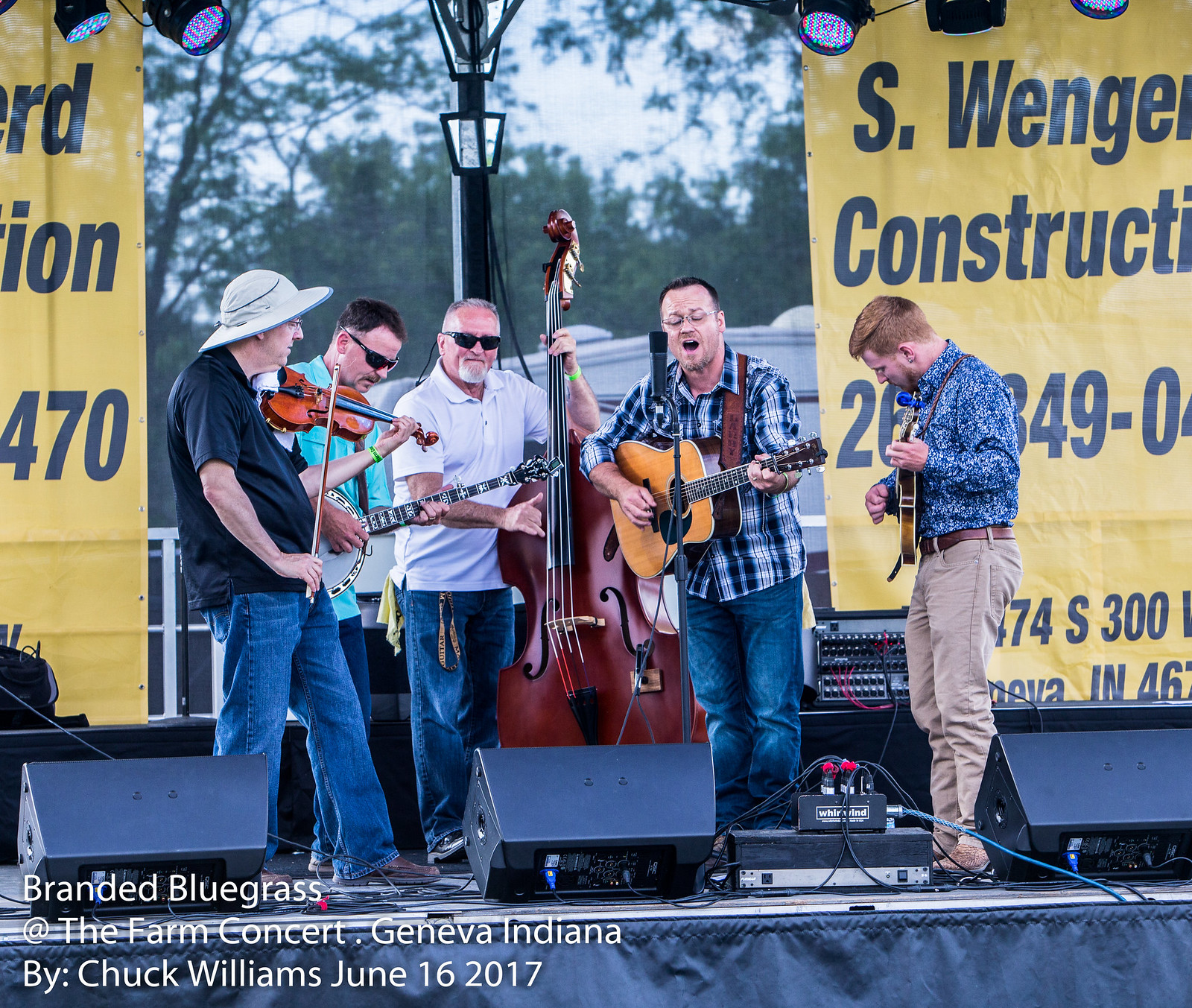This photograph, taken at an outdoor concert on June 16th, 2017, titled "Branded Bluegrass at the Farm Concert" in Geneva, Indiana by Chuck Williams, features five men, seemingly mature in age with a couple appearing slightly younger. They are assembled on a stage with three speaker monitors in front of them, playing various musical instruments. The man at the center, who stands out in a white shirt and blue jeans, is holding a wooden upright bass. To his right, a man in khaki pants and a blue multicolored shirt plays a guitar. Another man to the right, dressed in a plaid shirt and jeans, sings while playing a guitar. On the far left, a man wearing a beige hat, black shirt, and green pants, later corrected to blue pants, is playing a violin. Beside him, a man in a bright blue shirt and jeans, sporting sunglasses, is playing a banjo. The backdrop includes two yellow panels promoting "S. Wenger Construction," with a building, a post, and an RV visible in the distance, set against a background of distant trees. Fancy equipment including amplifiers are also part of their setup, hinting at the event's sophisticated arrangement.